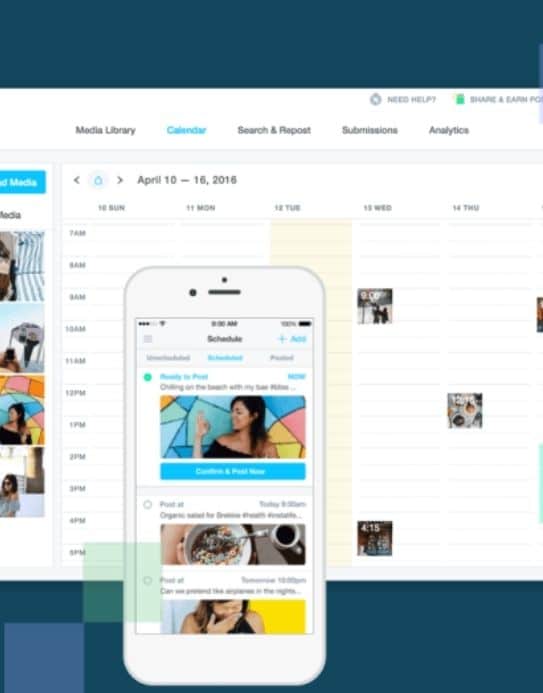The image showcases a calendar interface with a sleek design. The top and bottom borders of the image are adorned with a blue banner. The main section features a calendar with a white background and a light gray header, displaying the week from April 10th to 16th, 2016. The days of the week are labeled at the top: "10 Sun," "11 Mon," "12 Tue," "13 Wed," and "14 Thu."

Along the left side of the calendar, hours are listed vertically in hourly increments, starting from 7 AM and ending at 5 PM. Within the calendar grid are various small, almost JPEG-like images marking certain events or activities.

At the top of the interface, there is a set of clickable tabs for navigation: "Media Library," "Calendar," "Search," "Report," "Submissions," and "Analytics." The "Calendar" tab is highlighted in light blue, indicating it has been selected. To the upper right, there are buttons for "Need Help" and "Share and Earn Points."

Along the left vertical edge of the interface, four social media icons are partially visible, suggesting further integrations. Additionally, a "phone pop-out" overlay appears within the calendar, displaying several thumbnail pictures, indicating more detailed content or events linked to this specific date range.

Navigation arrows are present on either side of the calendar header to switch between different months, providing an intuitive way to browse through dates. Overall, the image depicts a well-structured and interactive calendar interface designed for efficient time management and event organization.